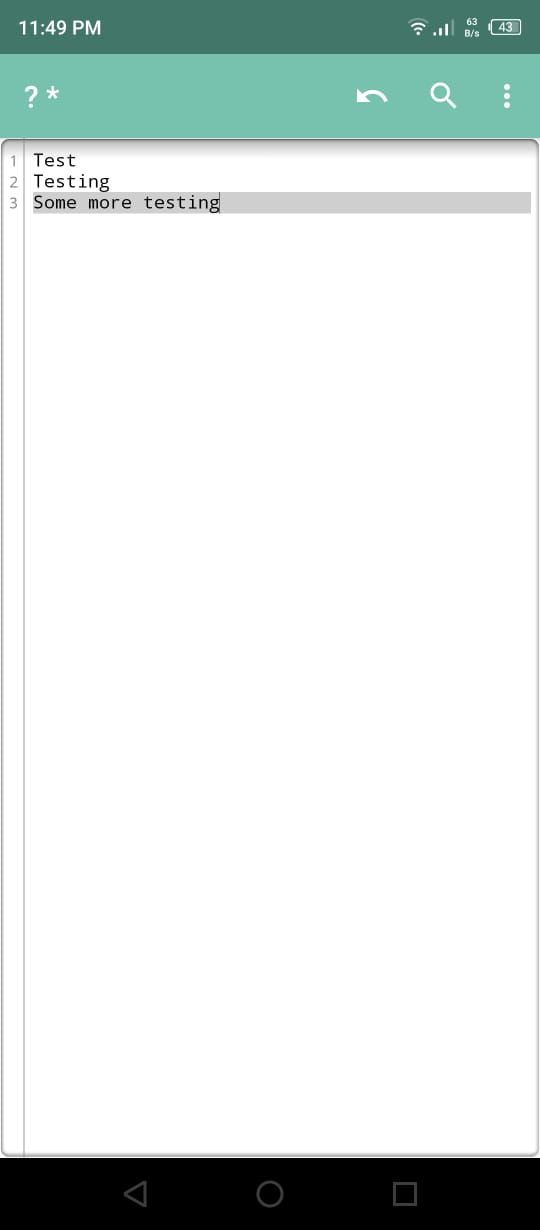This image showcases a coding app user interface displayed on a smartphone screen. In the header section, which features a green background, there are icons in white: a question mark and a star on the top left, and three buttons (redo, search, and a vertical three-dot menu) on the top right. The main content area has a white background and contains three lines of code, each numbered one to three. The numbers are in gray while the code text is in black. The lines of code read as follows: 
1. "test" 
2. "testing" 
3. "some more testing"

The third line is additionally highlighted in gray. At the bottom of the screen, standard navigation buttons can be seen, including back, minimize, home, and reset buttons. This comprehensive layout offers both functional and visual clarity for coding activities on the go.